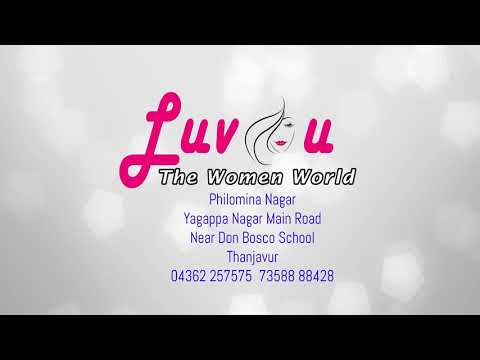The image is an advertisement with a light blue and white background, featuring a subtle circular white design, perhaps suggesting light. Across the top and bottom, there are thick black rectangular borders running horizontally. The prominent text, "Love You," uses a creative font where the letters 'OU' incorporate a drawing of a woman's face, symbolizing the 'O,' with flowing hair covering her left eye and she is depicted wearing lipstick; the 'U' is in pink. Below this, "The Women's World" is written in white font against a black background. Subsequent details include the text "Philomena Nagar, Yagapa Nagar, Main Road, near Don Bosco School, Sanjaver," all in purple or blue font. The contact number displayed is "04362-257575 73588 88428," with spaces between the number groups for clarity.